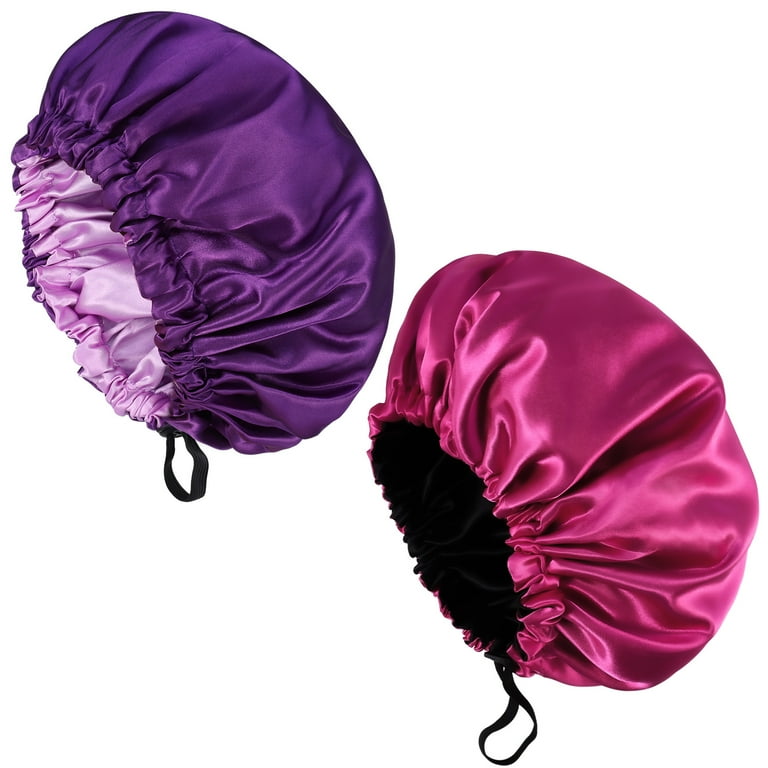The photograph features two sleek and shiny hair bonnets displayed against a white background. Both bonnets are made from a slick, silky, satin-like fabric that gleams under the light, highlighting the luxurious texture. Each bonnet has an elastic edge, creating pleats and wrinkles that reveal the reflective quality of the material. One bonnet, positioned higher in the image, showcases a dark royal purple exterior with a contrasting pink interior. The other bonnet, positioned slightly lower to the right, has a dark pink exterior with a black interior. Both have a small black string or loop at the bottom edge, likely for tightening or hanging the bonnets. These hair accessories are designed to protect hair from frizz and damage, typically worn overnight to keep hair smooth and secure. The bonnets appear to be identical in size and are oriented to the left, as viewed in the image.